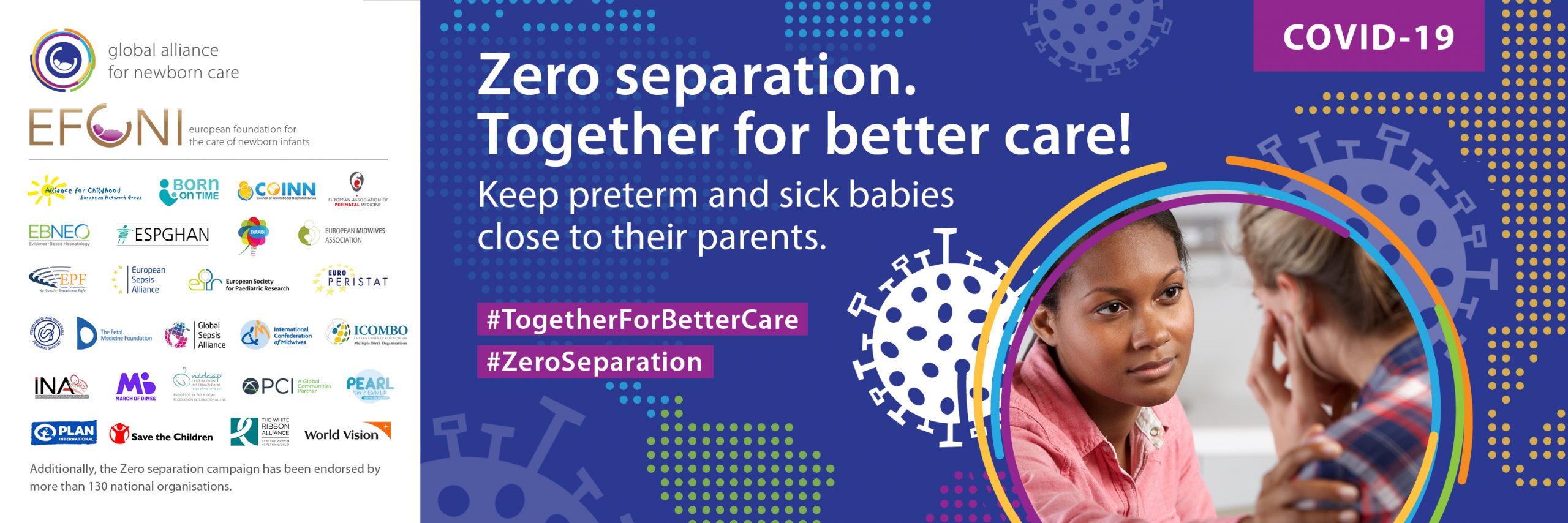**Banner Advertisement: "Global Alliance for Newborn Care"**

Left Section:
- A smaller, square, white section filled with an assortment of logos.
- Top text reads: "Global Alliance for Newborn Care."
- Midsection contains the acronym "EFONI," with a detailed explanation to the right in very small text.
- Beneath the logos, additional explanatory text in a tiny font.

Right Section:
- Features a blue background with a dotted design, possibly representing bacteria or another medical element.
- Prominent text reads: "Zero separation: together for better care. Keep preterm and sick babies close to their parents," followed by hashtags: "#ForBetterCare" and "#ZeroSeparation."
- To the right within a circular border, an image shows two women:
  - The woman on the left gazes at the other with concern and compassion.
  - The second woman presents her back to the viewer.
- Above the image of the women, the text reads: "COVID-19."